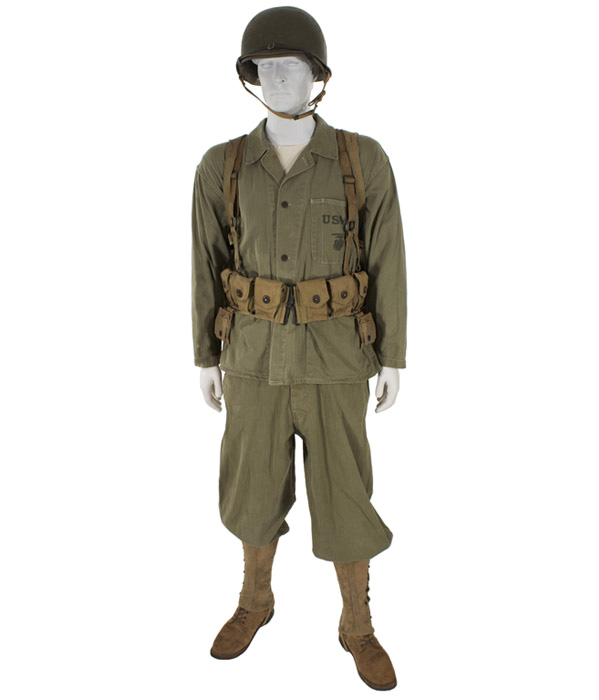This image captures a white male mannequin dressed in a historical U.S. Army uniform, likely from the World War II era, although some elements like the spats suggest it could be as early as World War I. The mannequin is posed in an 'at ease' position against a completely white background, enhancing the focus on the uniform itself.

The head is adorned with a typical steel pot olive drab helmet, securely fastened under the chin. The torso is covered in a long-sleeve, button-down green top with a collar and a visible pocket on the right chest area, partially covered by straps, but displaying the letters "U.S.A." There may be an insignia, possibly of a helicopter, on the pocket.

Straps extend over each shoulder, likely part of a web gear system, supporting an ammo belt encircling the waist. This belt comprises multiple rectangular pouches with fasteners, suggesting they may hold ammunition. Below this, the mannequin wears loose, baggy green pants that are not camouflaged. These pants are tucked into spats, a distinctive feature hinting at an older military uniform style, which are fastened and cover brown boots. The detailed construction of this uniform, with its various pouches and accessories, offers a thorough representation of a U.S. Army soldier's gear from an earlier conflict era.